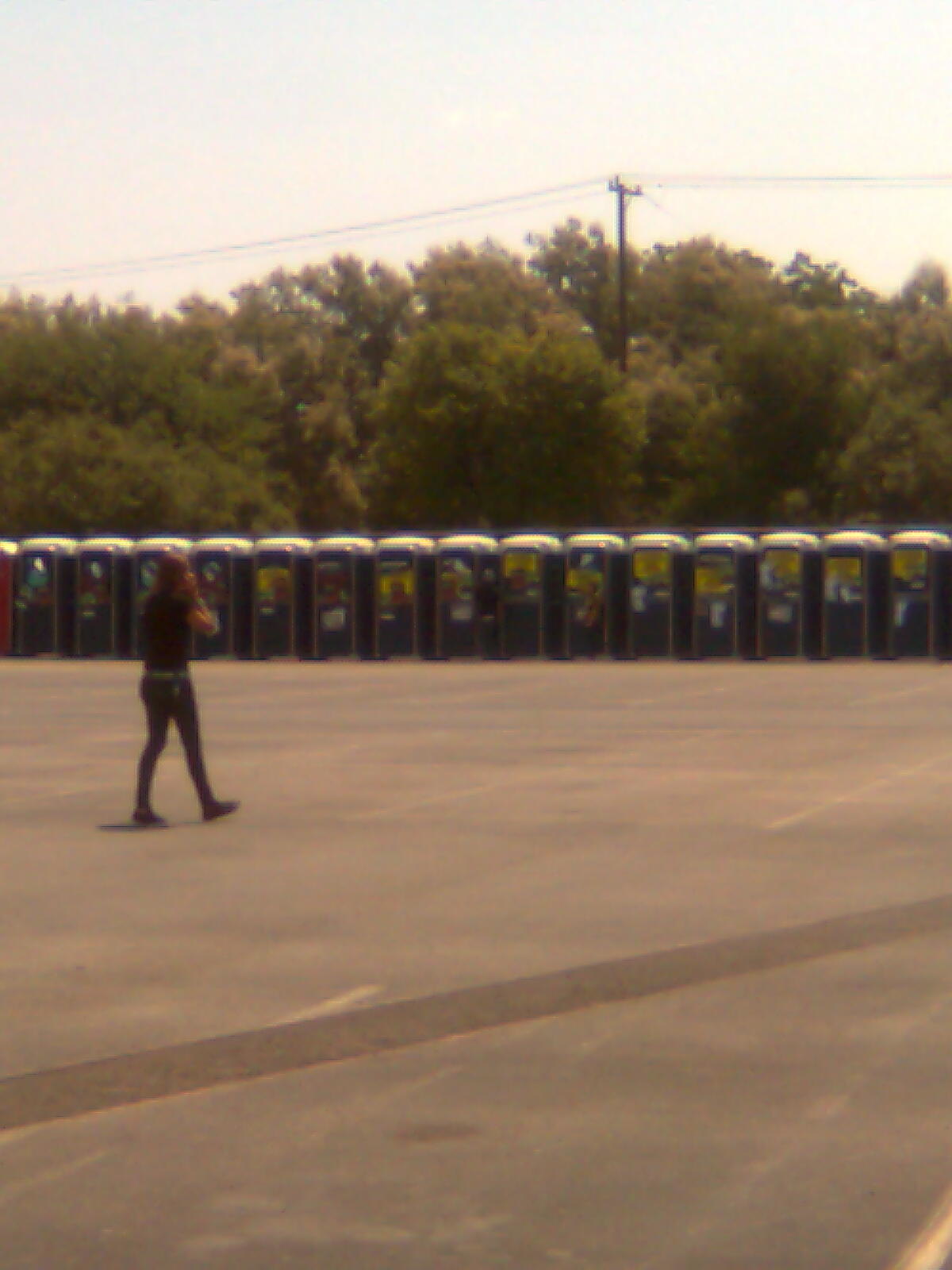This photograph appears to be an older, amateur, and low-quality image, characterized by a grainy and blurry texture. The scene is set outdoors in an empty, grey concrete parking lot with faded yellow and white lines delineating the parking spots. A person with long wavy brown hair, dressed in a black shirt and blue jeans, and potentially talking on a cell phone, walks across the lot from left to right, heading toward a prominently featured row of 18 blue porta-potties. Each porta-potty has a distinct yellow sign on its door and white tops. In the background, there is a dense forest of tall, green trees with an electrical power line running across the area. The overcast, grayish-white sky looms above, adding to the overall muted and dated feel of the photograph.